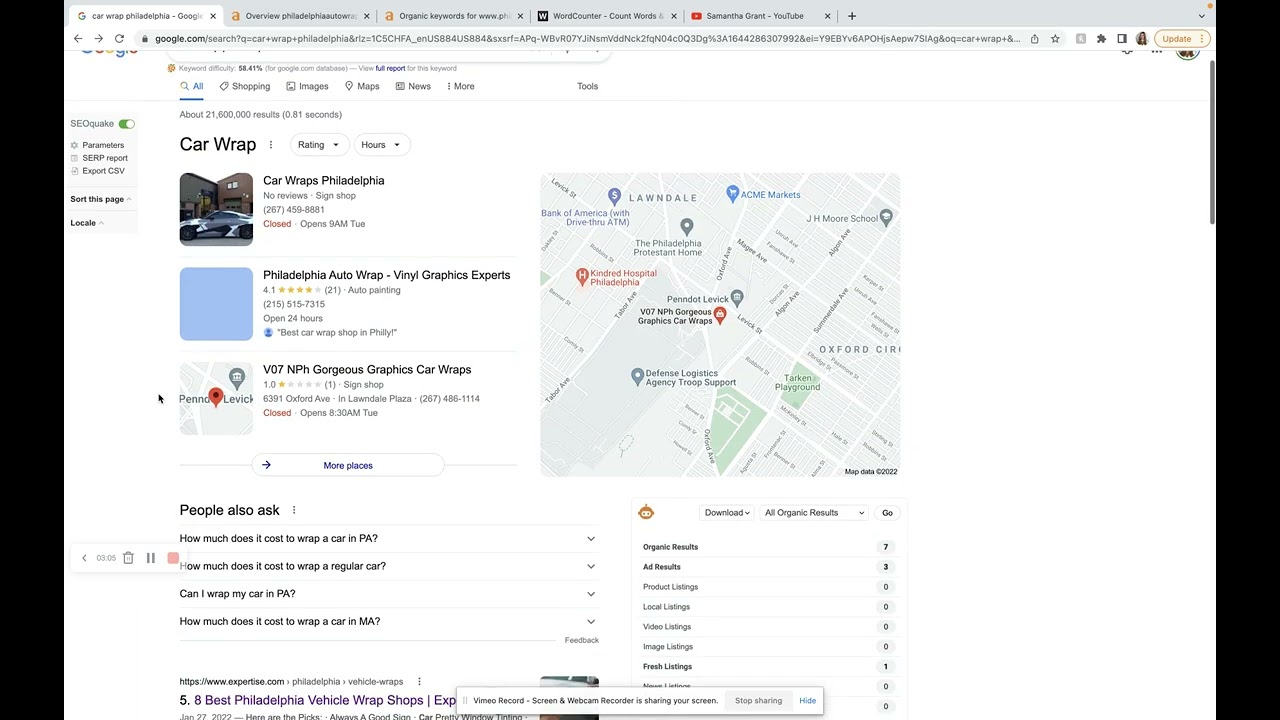The image displays a computer screen featuring a website. At the top of the screen, five tabs are open in the browser. Below the tabs, there is a URL search bar filled with the address "google.com" followed by a mix of letters, numbers, and additional text. 

Displayed prominently on the screen are search results for "Car Wraps Philadelphia." This includes various sections such as "All," "Shopping," "Images," "Maps," "News," and more. At the top of the results, there is a small square image of a wrapped vehicle with the title "Philadelphia Auto Wrap Vinyl Graphics Experts." Below the image, there is a description and contact information that includes a phone number for Philadelphia Auto Wrap. 

Positioned in the middle of the webpage is a map, presumably showing the Philadelphia area, indicating the location of the auto wrap service provider. The map provides a visual reference for the business's geographical context within the city.